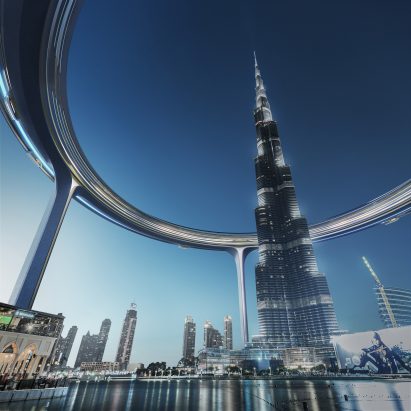The photograph captures a surreal cityscape dominated by a strikingly tall skyscraper with a pointed tip, its layered tiers giving it a futuristic, needle-like appearance. The skyscraper is adorned with scattered white lights, further enhancing its prominence against the gradient sky that transitions from dark blue at the top to lighter blue closer to the bottom left corner. Surrounding this colossal structure is a massive, circular monorail-like system, suspended on towering gray pillars, resembling the rims of a car tire. Below this architectural marvel lies a large, man-made lake that mirrors the city's skyline, adding depth and intrigue to the scene. In the bottom right, a large billboard with a white background displays a drawing of someone seated in a leather outfit. The combination of natural and artificial lighting, as well as the reflection on the water, creates an almost sci-fi atmosphere, making the scene reminiscent of a futuristic metropolis akin to something one might expect to find in Dubai.